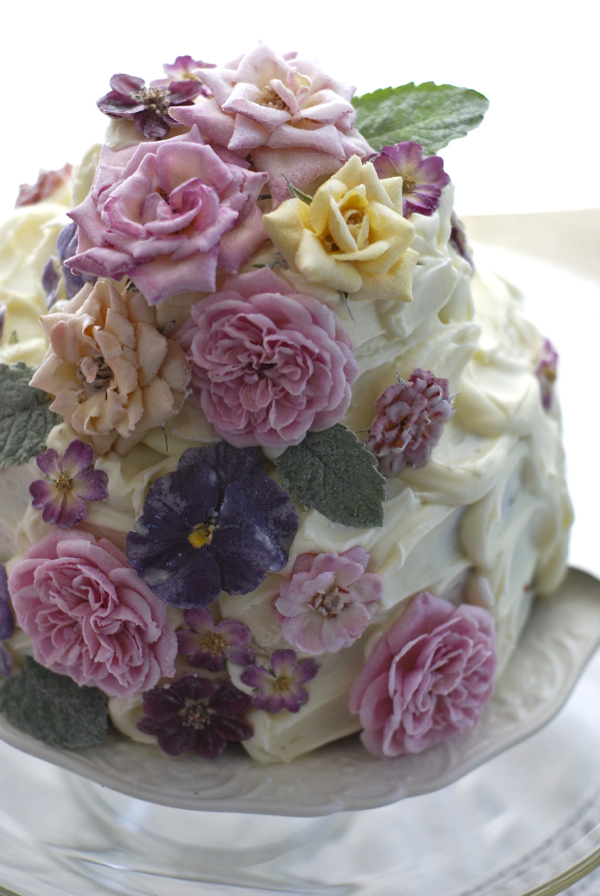This image features an elegant two-tiered wedding cake, resting on a white table adorned with a piece of crisp white cloth. Both tiers are covered in pristine white frosting, contributing to the overall white theme, which is enhanced by a stark white background. The bottom tier, larger in diameter, supports a slightly smaller top tier, creating a classic cascading structure.

The cake is tastefully decorated with an array of real flowers. The floral arrangement includes vibrant pink and yellow roses, along with darker and lighter purple rose-like flowers, adding a touch of color and elegance. The flowers are predominantly clustered on the left side of the cake, while the right side remains more minimalist, featuring just the smooth, white frosting. Additionally, green leaves, resembling those from a rosebush, are interspersed among the flowers, enhancing the natural and fresh look.

The top tier is adorned with pink, yellow, and blue flowers, as well as smaller purple flowers and a green leaf in the right corner. This careful placement of the floral elements creates a balanced and visually appealing design, making the cake suitable for various celebrations, such as weddings or possibly events with a feminine flair, like Mother's Day. However, without any candles or specific writing, the exact occasion remains open to interpretation, leaving it clear that this is a cake designed for a special, significant event.